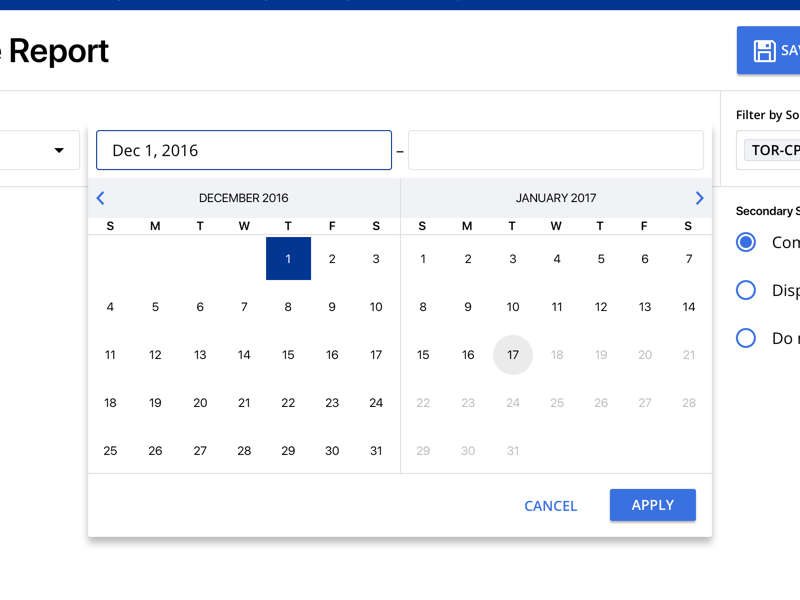The image depicts a detailed user interface of a calendar filtering tool. The background is predominantly white with a solid blue bar at the top displaying a partially cut-off label ending with "Report." To the right, there is a blue "Save" button featuring a floppy disk icon, but part of the label is also truncated, reading "Save."

Directly below this, there is an additional filtering option labeled "Filter by SO," with an input field currently set to "tor-cp." Further below, options labeled as "Secondary" filters are displayed with radio buttons: the selected one is "Con," while the other two options "Disp" and "Do" are available but not selected. These labels are also partially obscured.

The calendar interface is set to December 1st, 2016, highlighted with a blue box. An adjacent panel shows a partial view of January 2017, with a gray circle around January 17th, likely indicating the final date for applying the filter. Dates from January 18th to 31st are grayed out, distinguishing them from the selectable black dates.

Finally, there are two action buttons towards the bottom: a "Cancel" button and an "Apply" button, the latter prominently rendered in blue with white text.